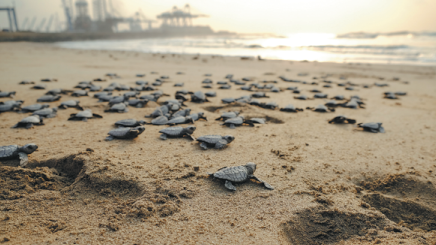In this vibrant, outdoor image captured during what appears to be either sunrise or sunset, we see hundreds of small, gray baby sea turtles scurrying across a wet, brown sandy beach towards the water on the upper right side of the picture. The turtles, identifiable by their little gray flippers and big black eyes, have just hatched and are instinctively making their way to the ocean to start their lives. The wet sand, embedded with grooved tracks from where the turtles emerged, adds texture and depth to the scene. In the background, to the upper left, there are some structures resembling canopies or buildings with roofs supported by pillars. The sky, painted with hues of orange, suggests the gentle transitioning time of day, either dawn or dusk. The distant shoreline and softly crashing waves beckon the tiny reptiles, while further in the distance, blurred shapes hint at larger constructions, possibly oil rigs or a naval base. The absence of people keeps the focus entirely on the turtles and their remarkable journey.